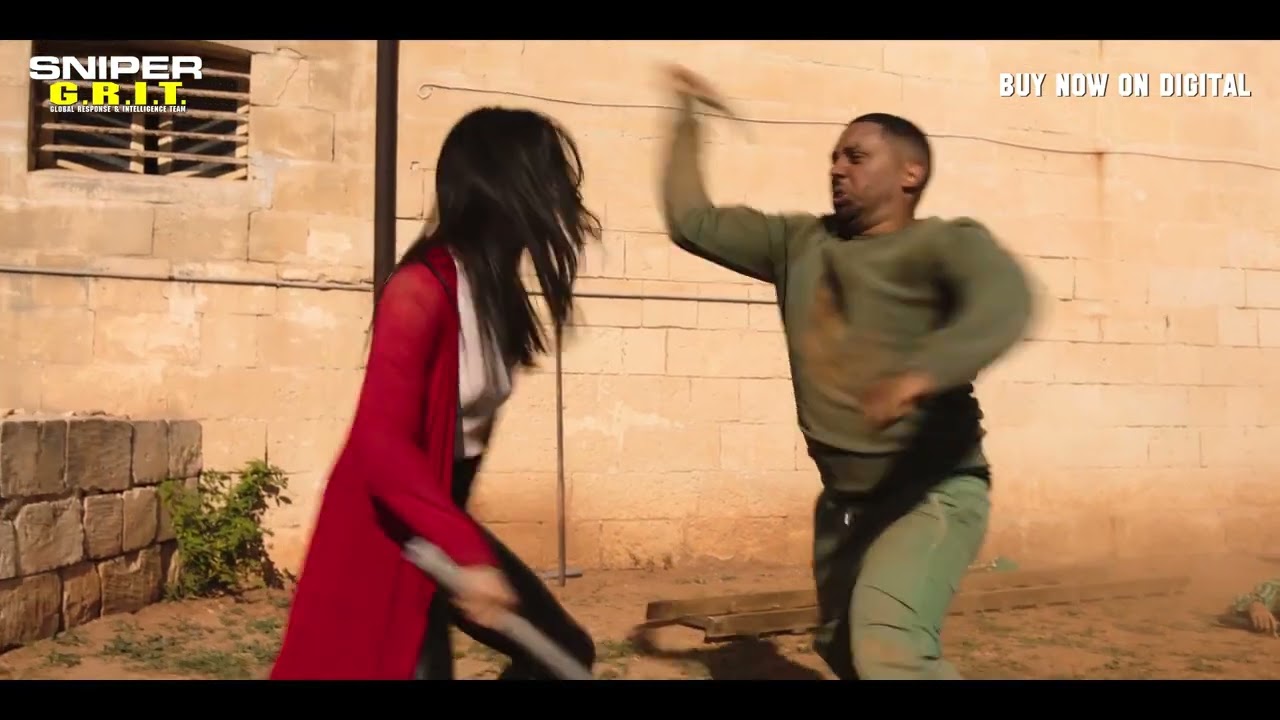In this image, we observe a high-resolution still from an action movie or an advanced video game, contained within a rectangular frame where the top and bottom are longer than the sides. Overlaying this image are two solid black banners running across the top and bottom edges, each approximately three-quarters of a centimeter in height. The background reveals two adjoining walls, constructed from large bricks composed of smaller horizontally-aligned bricks, all in a pinkish-peach color. A centimeter gap separates these walls. On the top left portion of the image, there's a rectangular window with horizontal slats or bars, through which sunlight streams. Above this window, in the top left corner, the text "SNIPER" appears in white, all-caps lettering, and directly beneath it in yellow, all-caps, reads "GRIT" (possibly an acronym for "Global Response and Intelligence Team").

In the foreground, a woman with silky black, shoulder-length hair that obscures part of her face is seen. She wears a white shirt, a long red cardigan, and black pants. Her right arm is bent at the elbow, holding a stick-like object at a diagonal angle. Facing her is a man, whose torso is turned slightly towards her, wearing a dirty olive green long-sleeve shirt and matching green pants. His right arm, also bent at the elbow and motion-blurred, suggests he may be striking or defending against the woman. He has a short, faded haircut. Additional scene details include a board or stick lying on the dusty, pinkish dirt ground near them, and sparse vegetation to the left.

In the top right corner, white, all-caps text reads "BUY NOW ON DIGITAL," suggesting promotional content. The action scene, coupled with the titular information and dynamic confrontation, implies a tense, possibly combat-intense moment in the narrative.